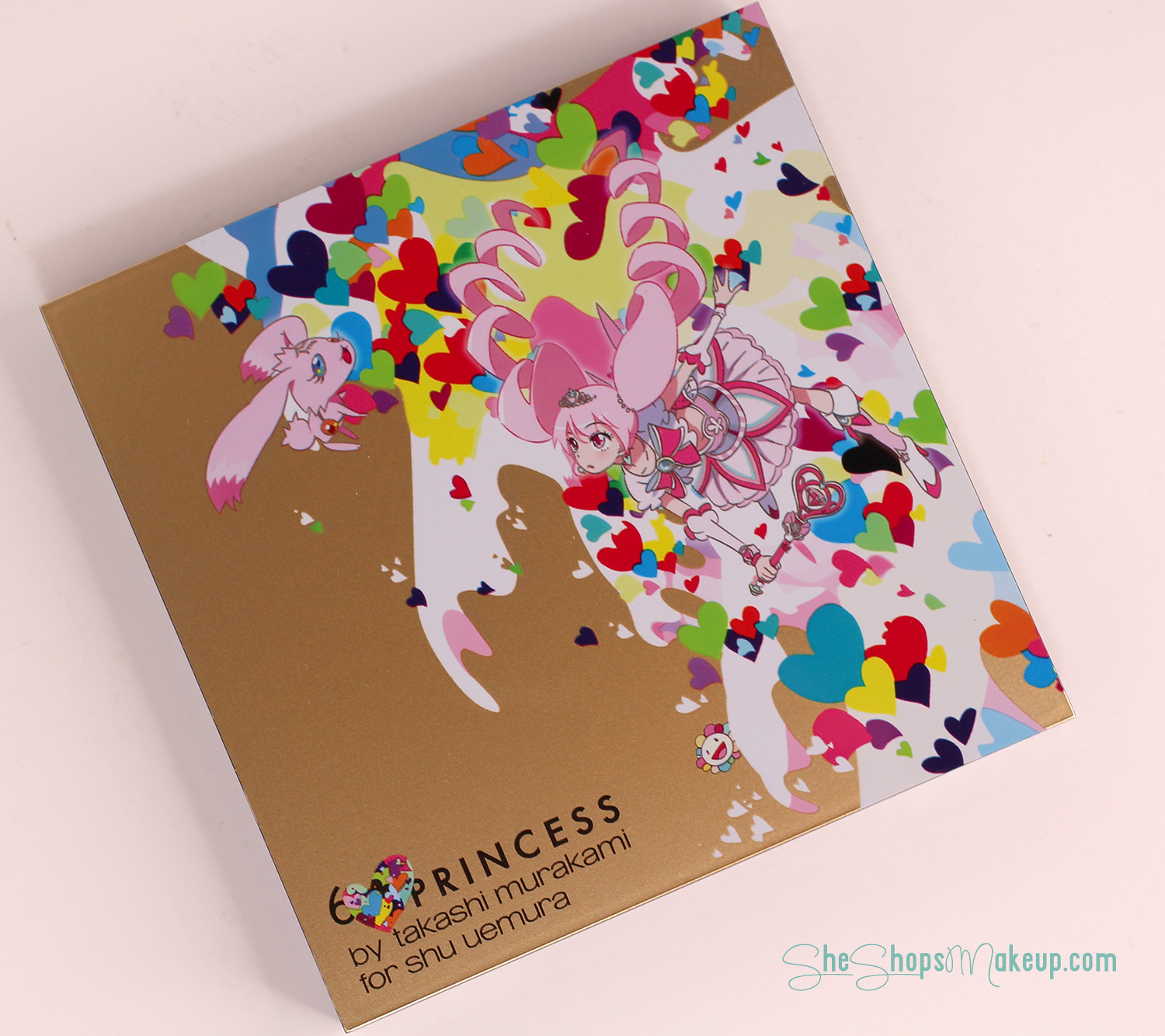The book cover image is set on a flat, faint light pink surface. Positioned at an angle, the cover's top right corner points towards the top of the image, while the bottom left corner points towards the bottom. On the bottom right of the cover, in blue text, it reads "SheShopsMakeup.com." 

The left side of the cover features a gold background, transitioning to a splash of white on the right side, adorned with multiple colored hearts including yellow, teal, green, purple, white, black, and red. In front of these colorful hearts, there is an anime cartoon-style girl holding a heart-shaped wand. She is dressed in a white dress with pink frills and a large pink bow on her chest. Additionally, there is a pink fairy and a flying pink animal with long ears featured in the artwork. At the bottom right of the box, in black text, it reads "Six Princess" by Takashi Murakami for Shu Uemura.